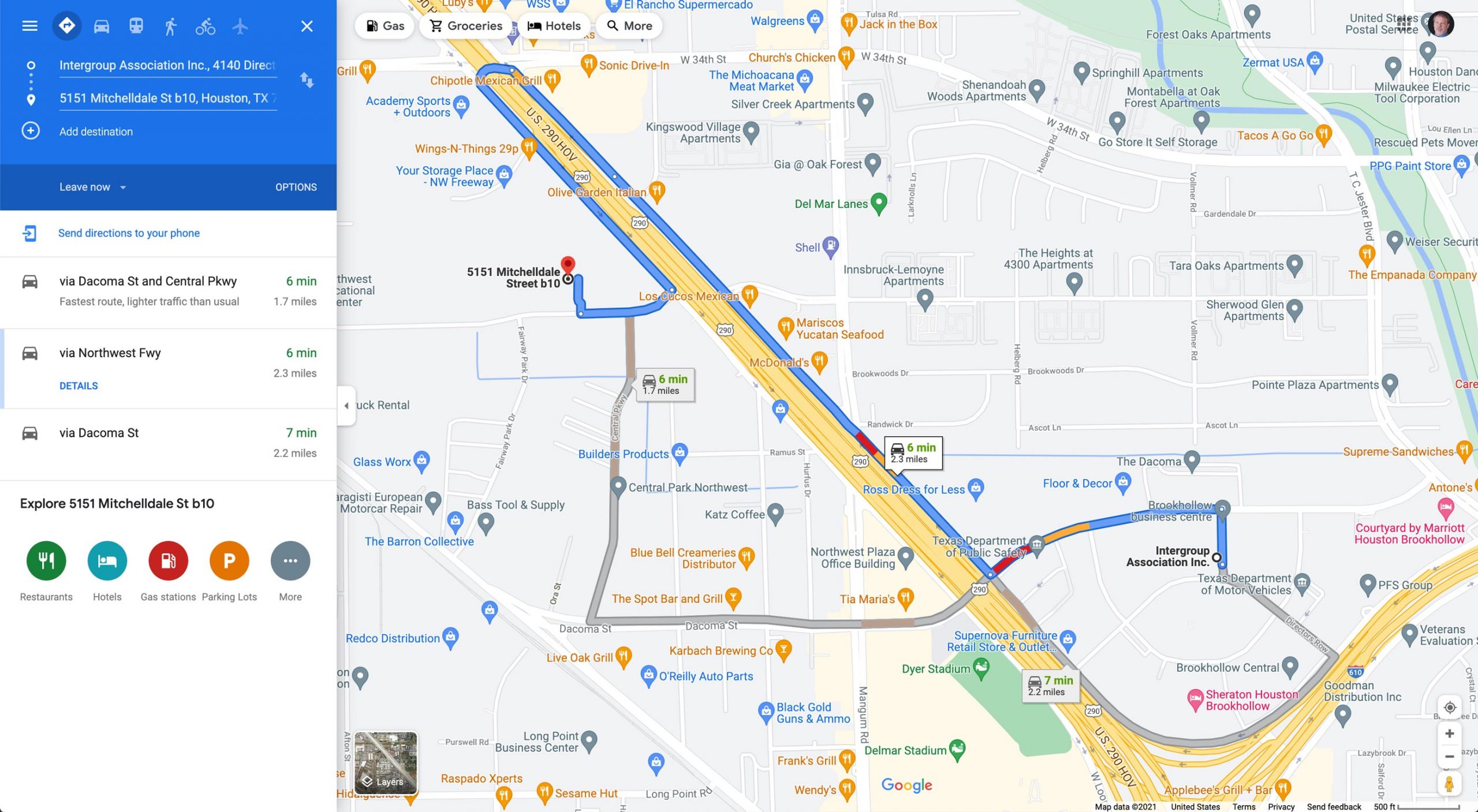This image is a screenshot from Google Maps showing detailed navigation instructions.

In the top right corner, a small circular icon displays a person’s profile photo, though details are indistinguishable due to its size. On the left side, the current navigation details are visible, indicating that directions are being sought from Intergroup Association, Inc., at 4140 (with the rest of the address cut off) to 5151 Mitchelldale Street, B10, Houston, Texas. Beneath the destination, the instruction to "leave now" is displayed, along with an option to send the directions to a phone.

Three different driving routes are provided. The fastest route, taking 6 minutes, follows Decoma Street and Central Parkway and is noted to have lighter traffic than usual. The second route, also 6 minutes, follows Northwest Parkway. The third route, taking 7 minutes, follows Decoma Street. Additionally, options to explore nearby amenities such as restaurants, hotels, gas stations, and parking lots are available.

The right side of the screenshot shows a 2D map with the route depicted in grey, while parks and green spaces are highlighted in green.